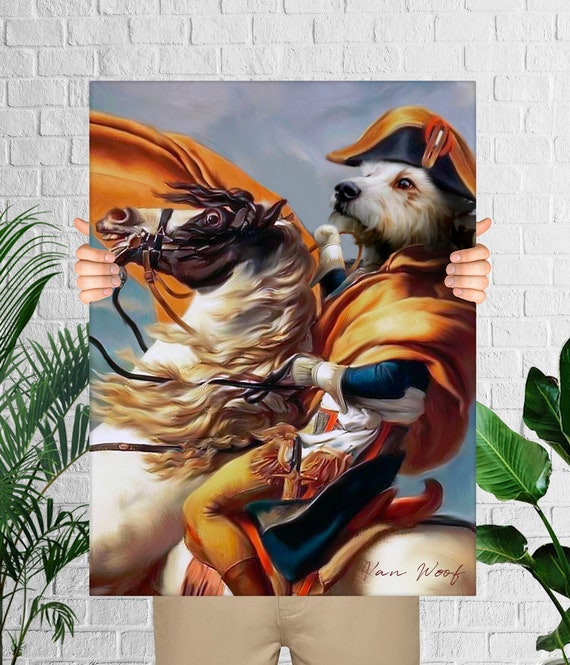In this image, a person, whose gender is indeterminate, stands in front of a white brick wall, holding a painting in front of their torso. Their tan slacks and white fingers are visible, as they grip the edges of the rectangular painting. The scene is flanked by green plants. The artwork portrays a dog, reminiscent of a terrier, dressed in a Napoleonic military outfit, complete with a gold and black hat and an orange and dark blue uniform. The dog, with tan legs and gloved paws, confidently rides a white horse with a goldish mane, a black and white face, and a brown eye. The horse's saddle appears red and brown. In the bottom right corner of the painting, the signature "Van Woof" is elegantly scripted in tan.